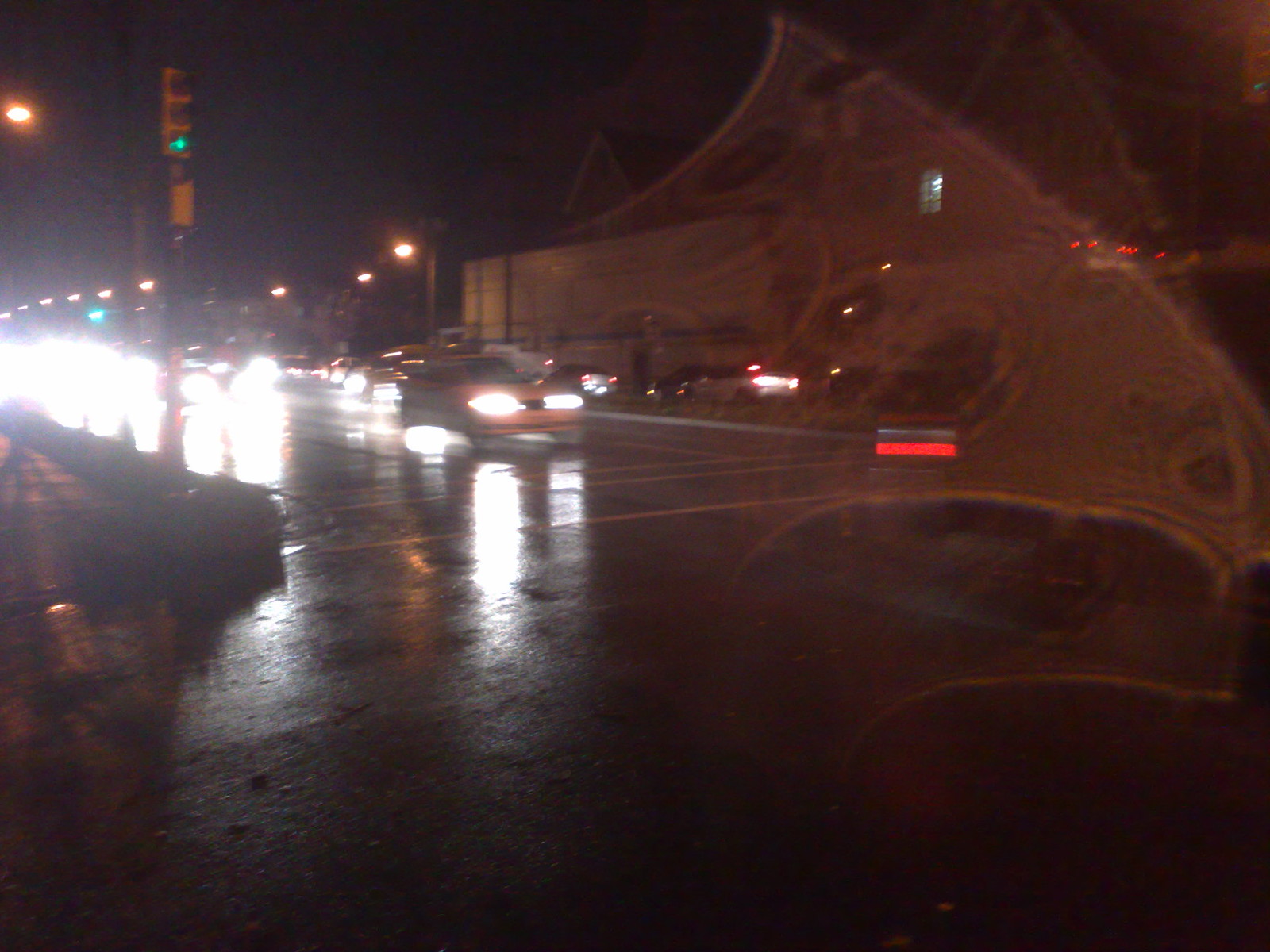The photograph captures a nighttime urban street scene, obscured by a noticeable haze or light glare that produces a blurry blob across the image. The wet pavement suggests recent rain, reflecting the bright headlights of numerous cars moving through the dark street. Towards the left side of the picture, the intensity of the car lights makes it difficult to discern individual vehicles. A white car is visible more distinctly among the traffic. The upper part and background of the image reveal a large building and perhaps a house, illuminated slightly by a green streetlight on the left and another light source on the top right from a nearby structure. The overall dark, wet atmosphere is further accentuated by reflections and possible motion blur, indicating the image might have been taken from inside a moving vehicle. The scene offers a stark contrast with glaring lights piercing through the dark, rain-soaked setting, rendering the night both vibrant and obscure.